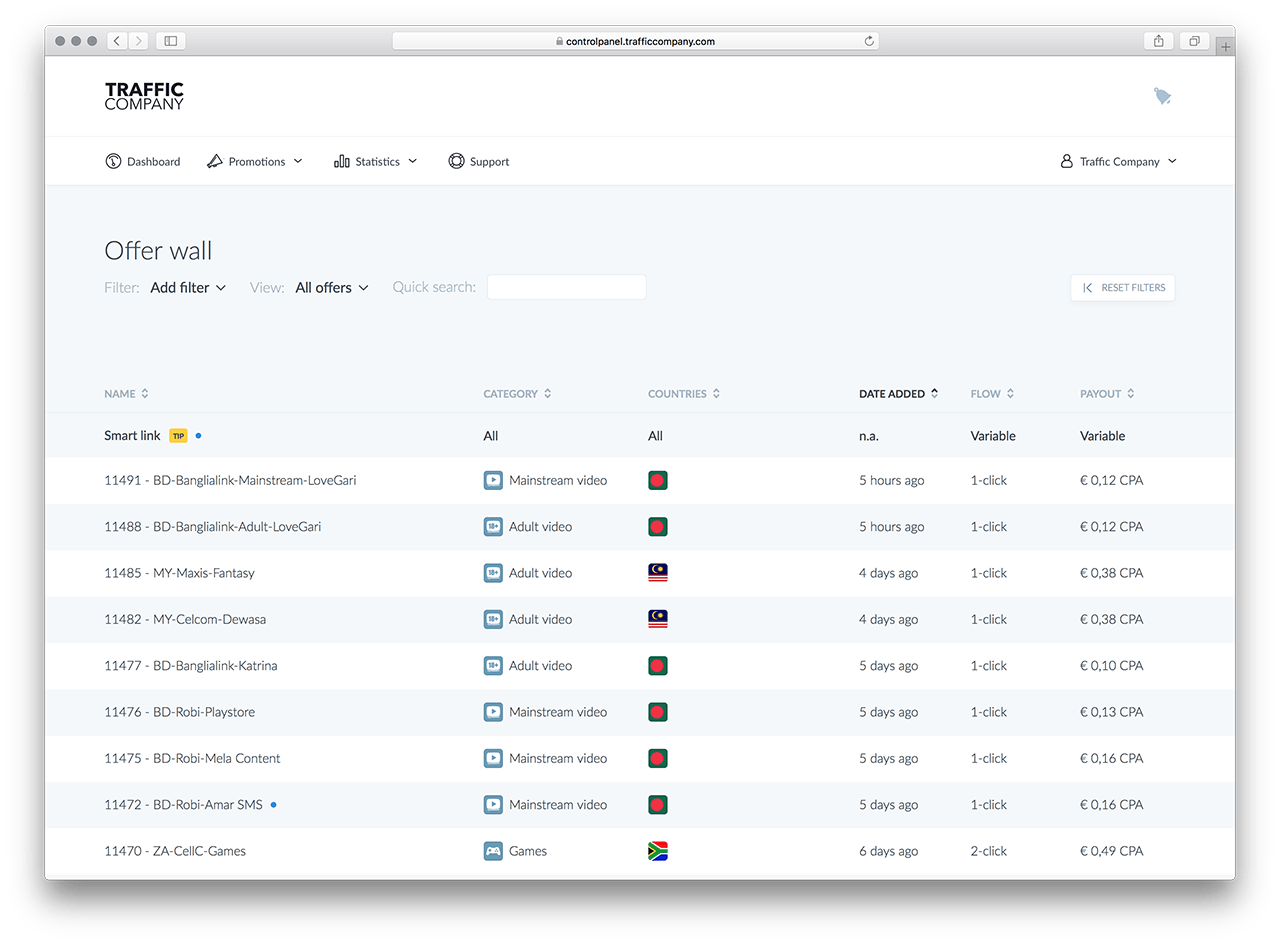**Detailed Screenshot Description of Website within a Browser**

The image captures a detailed screenshot of a browser window displaying a website. The browser window features an outlined border with a noticeable shadow effect around it. 

At the very top of the browser, there is the standard browser bar:
- On the left-hand side, there are three circular dark gray icons typically used for window control (e.g., minimize, maximize, and close).
- Next to these icons, the back and forward navigation buttons are present but grayed out, indicating they are not currently usable.
- A small indistinguishable icon sits to the right of the navigation buttons.

Centrally located in the top bar is the URL bar:
- This bar contains a padlock icon followed by the website's URL, which is too small to read clearly.
- The URL bar has a white background with black text.
- On the far right of the top bar are a few additional, unspecified icons.

The main content area of the browser displays the website:
- The header section spans the width of the screen and has a white background.
  - In the top-left corner, the logo reads "Traffic" in bold, followed by "Company" in non-bold text beneath it.
  - In the top-right corner of the header, there's a gray bell icon that suggests notifications.
- Below the header, a space provides separation before leading to the main navigation bar at the bottom of the header.
  - The navigation options are listed from left to right as follows: 
    - "Dashboard" with a meter icon,
    - "Promotions,"
    - "Statistics,"
    - "Support."
  - On the far right, "Traffic Company" is presented with a drop-down menu icon and a small person symbol to the left of it.

A dividing line comes next, separating the header from the main content area below it.

Within the main body of the website, which has a light gray background, the content is as follows:
- The top section is labeled as "Offer Wall," with options for filtering, viewing, and a quick search.
- Below this heading is a series of approximately 10 rows representing a data list, structured into six columns:
  - The columns are titled "Name," "Category," "Countries," "Date Added," "Flow," and "Payout."
  - The first row appears unique, labeled with "Smart Link," "All" for both Category and Countries, "N/A" for Date Added, and "Variable" for both Flow and Payout.
- Subsequent rows follow a similar structure but with different entries:
  - The second row, for example, features "11491 BO Bargland Link something," categorized under "Mall Stream Video" with data such as "five hours ago" under Date Added and "one click" under Payout.
- The rows alternate in color from light to light gray, each accompanied by respective icons denoting various categories and countries.

This detailed structure blends a thorough visual walkthrough of the browser layout, header and navigation specifics, as well as granular content details within the website displayed.